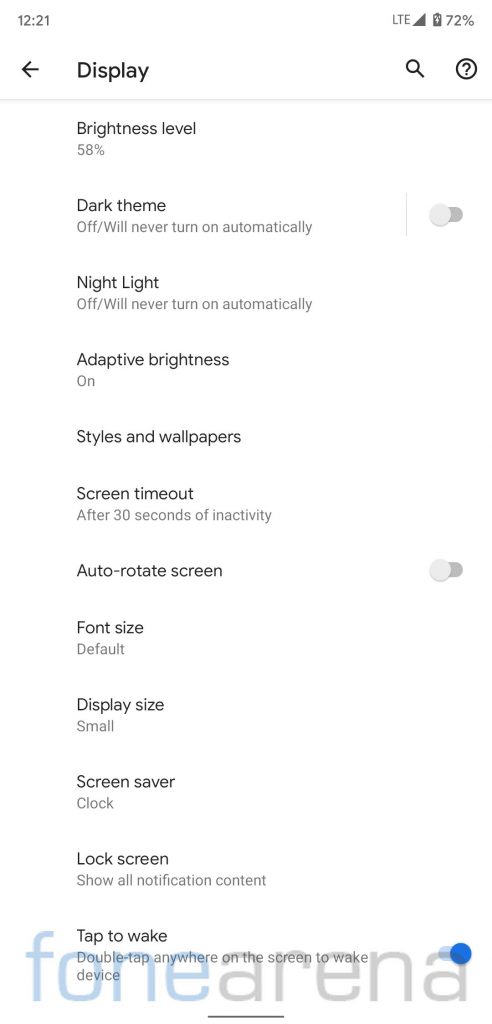The image depicts a screenshot of the display settings menu on an Android phone. The top portion of the screen is white, displaying various system indicators. In the top left corner, the time reads "12:21" in black text. To the right are symbols indicating an LTE connection with full signal strength (a black, filled-in triangle pointing downward) and a battery icon displaying "72%". 

Beneath these indicators is a header with a left-facing arrow labeled "Display", alongside a magnifying glass icon on the right and a question mark enclosed in a circle. 

The main body of the screen is divided into multiple settings options:

1. **Brightness level**: Set at 58%.
2. **Dark theme**: Displayed as "Off / Will never turn on automatically" with a gray toggle switch to the right.
3. **Night Light**: Indicated in bold, stated as "Off / Will never turn on automatically".
4. **Adaptive brightness**: Set to "On".
5. **Styles and wallpapers**: Listed without further detail.
6. **Screen timeout**: Configured to "After 30 seconds of inactivity".
7. **Auto-rotate screen**: Also equipped with a toggle switch.
8. **Font size**: Set to "Default".
9. **Display size**: Set to "Small".
10. **Screen saver**: Set to "Clock".
11. **Lock screen**: Configured to "Show all notification content".
12. **Tap to wake**: Enabled with a blue toggle switch, noted as "Double tap anywhere on the screen to wake device".

The detailed breakdown reveals various display settings, including brightness adjustments, theme preferences, and lock screen customizations, providing a comprehensive look at the phone's current display configuration.